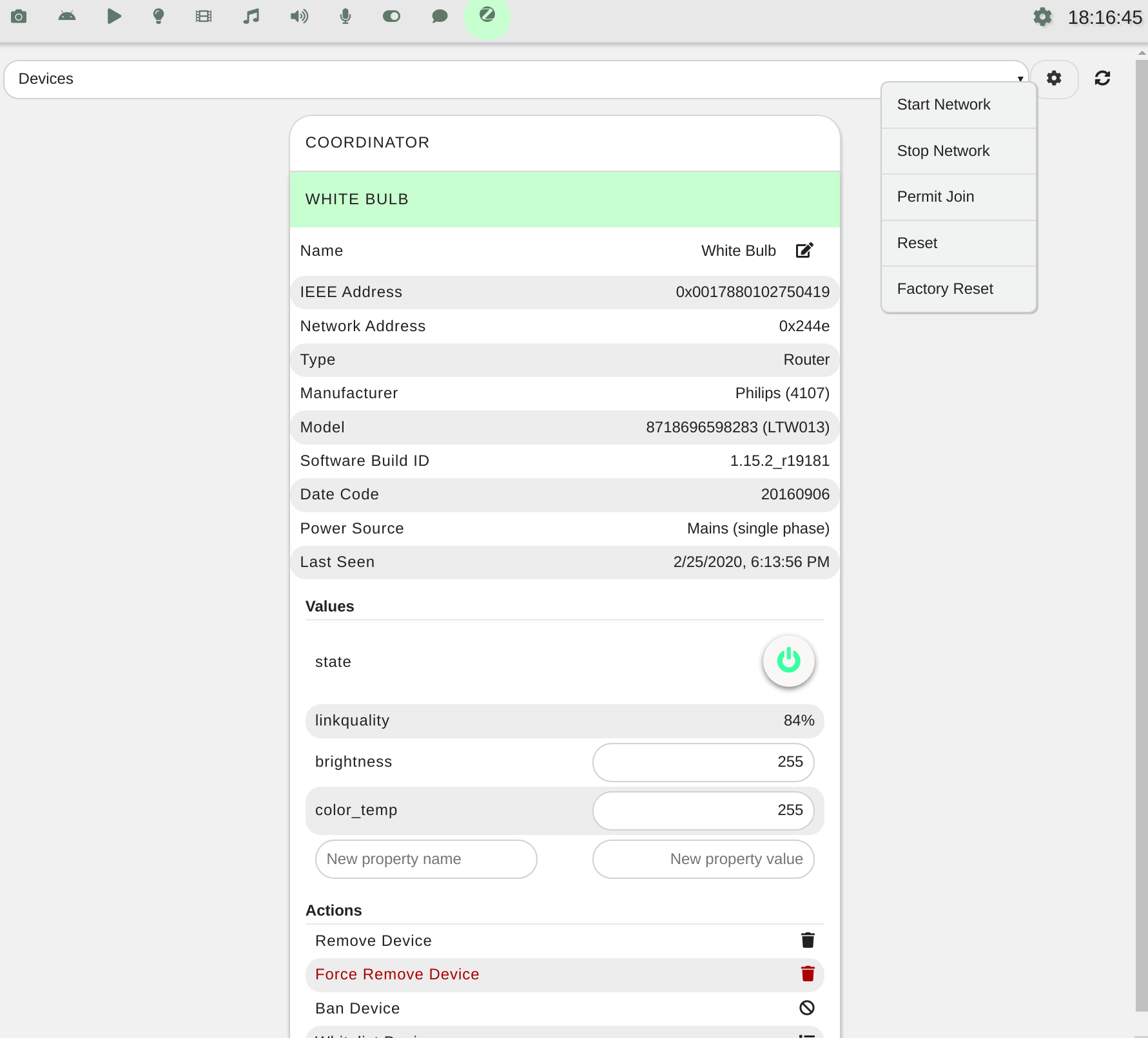The image depicts a user interface designed for managing smart devices, with a focus on controlling a smart light bulb. The header at the top displays the time in a detailed 24-hour format, showing hours, minutes, and even seconds, currently reading 18:16:45.

Within the header, various icons are visible, representing different functionalities. These include familiar symbols for Home, Play, Settings, a Light Bulb emblem likely indicating smart light controls or an FAQ/idea section, a Search function, a Music emblem, and several other icons that are not explicitly named.

The central section of the interface prominently features a segment labeled "DEVICE MANAGEMENT." Under this heading, "COORDINATOR" is displayed in all capital letters, indicating a central hub or main device that manages other connected devices. Beneath the "COORDINATOR" label, the text "WHITE BULB" is also written in capital letters and is highlighted in green, signifying that the smart light bulb is currently the device being managed.